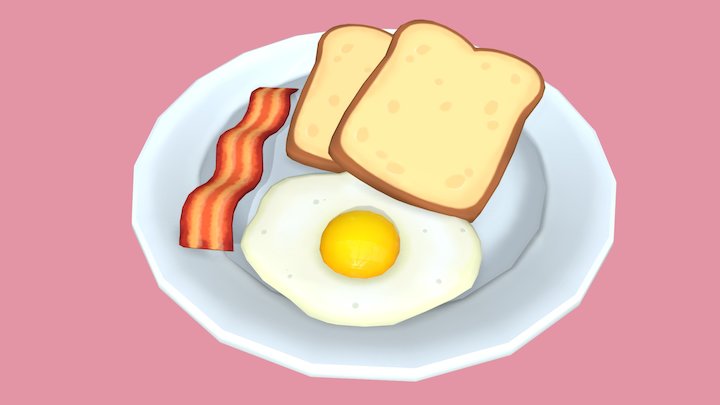The image depicts a hyper-cartoony breakfast scene set against a solid pink background. Centered on the jagged-edge white plate is a comical representation of classic breakfast items: a single, slightly undercooked strip of bacon with dark red edges and a pinkish midsection; a sunny side up egg with a disappointingly unappetizing appearance, resting deeply in the plate's middle impression; and two pieces of white toast stacked atop each other, showcasing numerous air pockets and holes. The entire arrangement, clearly the work of a professional cartoonist, is devoid of any text or utensils, emphasizing the exaggerated, non-realistic style of the artwork.